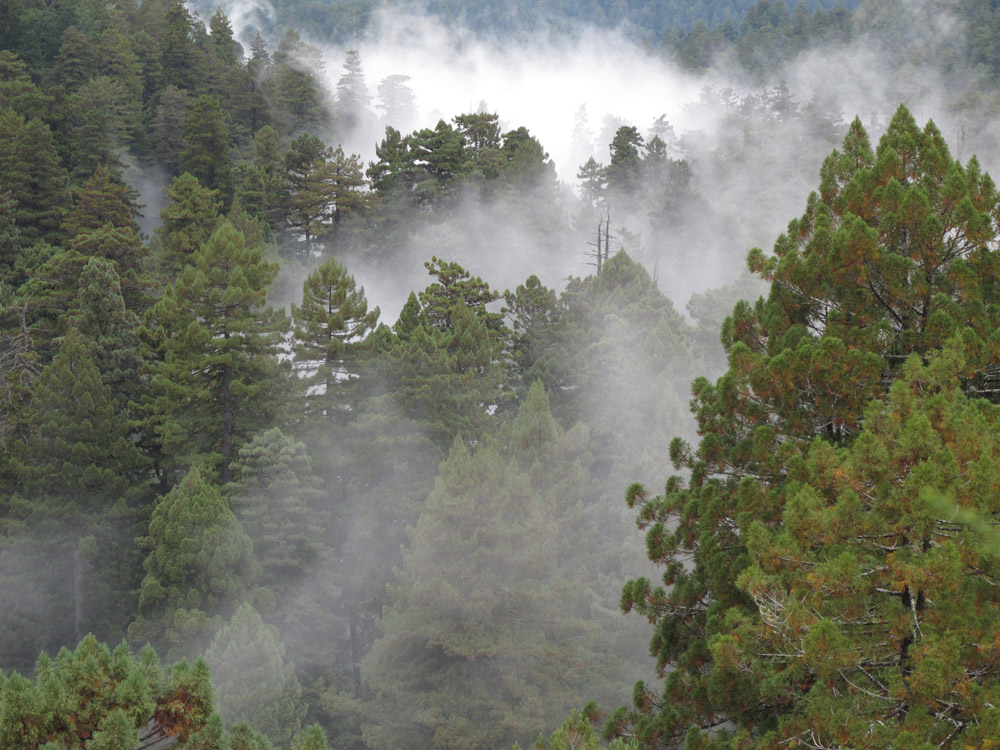The photograph captures a vast, lush forest from a high vantage point, possibly from a hill or elevated structure, providing a sweeping view above the treetops. The scene is vibrant with tall, green evergreen trees, their conical shapes distinct. A dense white mist or fog weaves through the forest, blanketing the greenery in layers. This mist is thicker and more opaque in the distant background, where the trees gradually fade into a hazy, out-of-focus expanse, suggesting the forest's vastness. Closer to the foreground, the mist thins, allowing the vivid green of the healthy trees to stand out more clearly. The atmosphere is serene and entirely natural, with no signs of human interference, capturing the pure essence of an expansive and thriving forest wilderness.